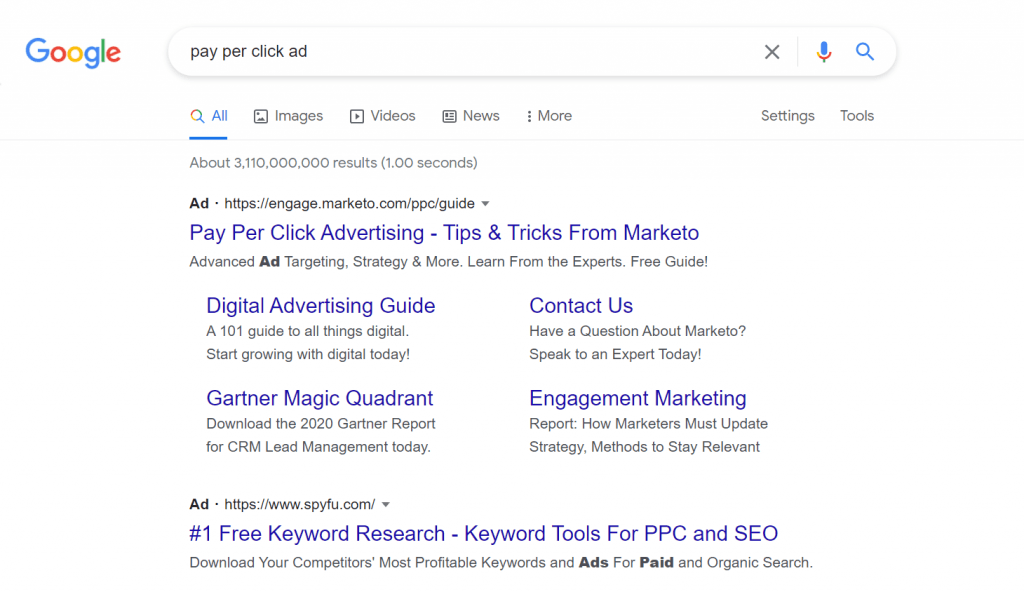In this image, a Google search has been performed for the term "pay per click ad." The screen displays a standard Google search results page with a white background and familiar blue link text. Notably, the first two links that appear are both advertisements, which adds a layer of irony to the situation. The first ad is titled "Pay Per Click Advertising - Tips and Tricks from Markito," where "Markito" appears to be a playful misspelling of "market." The second ad presents "Number One Free Keyword Search, Research, Keyword Tools for PPC and SEO," highlighting resources for both pay-per-click (PPC) advertising and search engine optimization (SEO). This juxtaposition humorously underscores the fact that even when searching for information about ads, users are, in turn, presented with more ads. The total number of search results is also visible, exceeding 3 billion, and reinforcing the vastness of information available online.